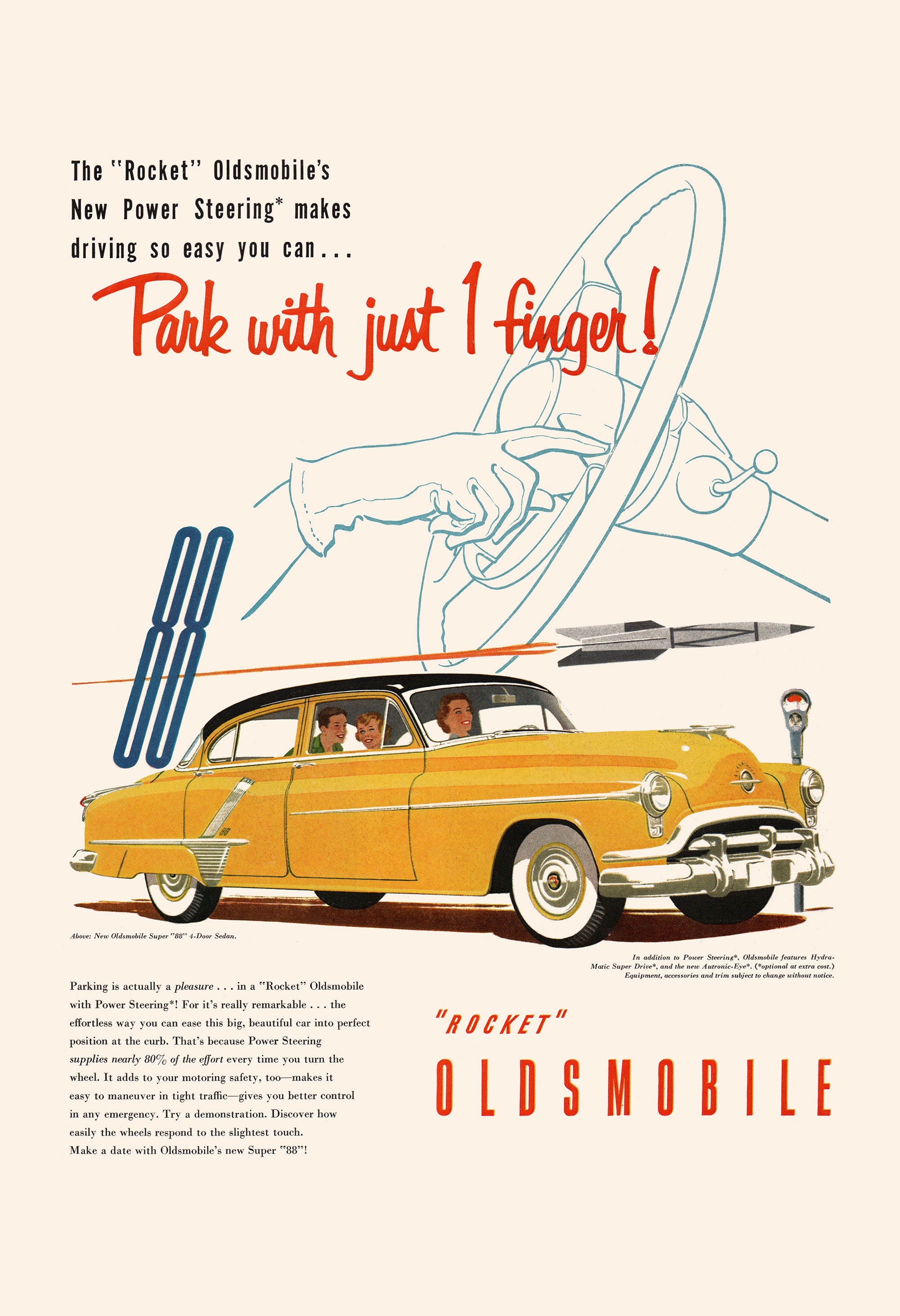This vertically-oriented vintage advertisement from the 1950s or early 1960s features a cream-colored background promoting the Rocket Oldsmobile's new power steering technology. Dominating the center is an illustration of a yellow four-door American car with a black hardtop and whitewall tires, hinting at the sleek, chrome-detailed designs of that era. The car, a Super 88 model, is parked next to a parking meter, and inside, a smiling woman is at the wheel while two children sit in the back seat.

At the top left of the poster, black lettering announces, "The 'Rocket' Oldsmobile's new power steering makes driving so easy you can..." In larger red letters below it continues, "park with just one finger." A blue-outlined sketch illustrates a woman's gloved finger effortlessly steering the wheel. A rocket graphic streaks across the top right, adding a sense of motion and excitement to the ad.

Towards the bottom, detailed text in smaller font extols the benefits of Oldsmobile's power steering, emphasizing the minimal effort required for parking and enhanced safety in tight traffic situations. The text reads, "Parking is actually a pleasure in a Rocket Oldsmobile with power steering, for it's really remarkable... the effortless way you can ease this big beautiful car into perfect position at the curb. That's because power steering provides nearly 80% of the effort every time you turn the wheel. It adds to your motoring safety too, makes it easier to maneuver in tight traffic, gives you better control in any emergency. Try a demonstration, discover how easily the wheels respond to the slightest touch. Make a date with Oldsmobile's new Super 88."

On the right side, additional text promotes other features such as Hydromatic Superdrive and the new Autronic Eye, emphasizing their optional availability and potential extra cost. The advertisement concludes with "Rocket Oldsmobile" in large, prominent red lettering at the bottom.